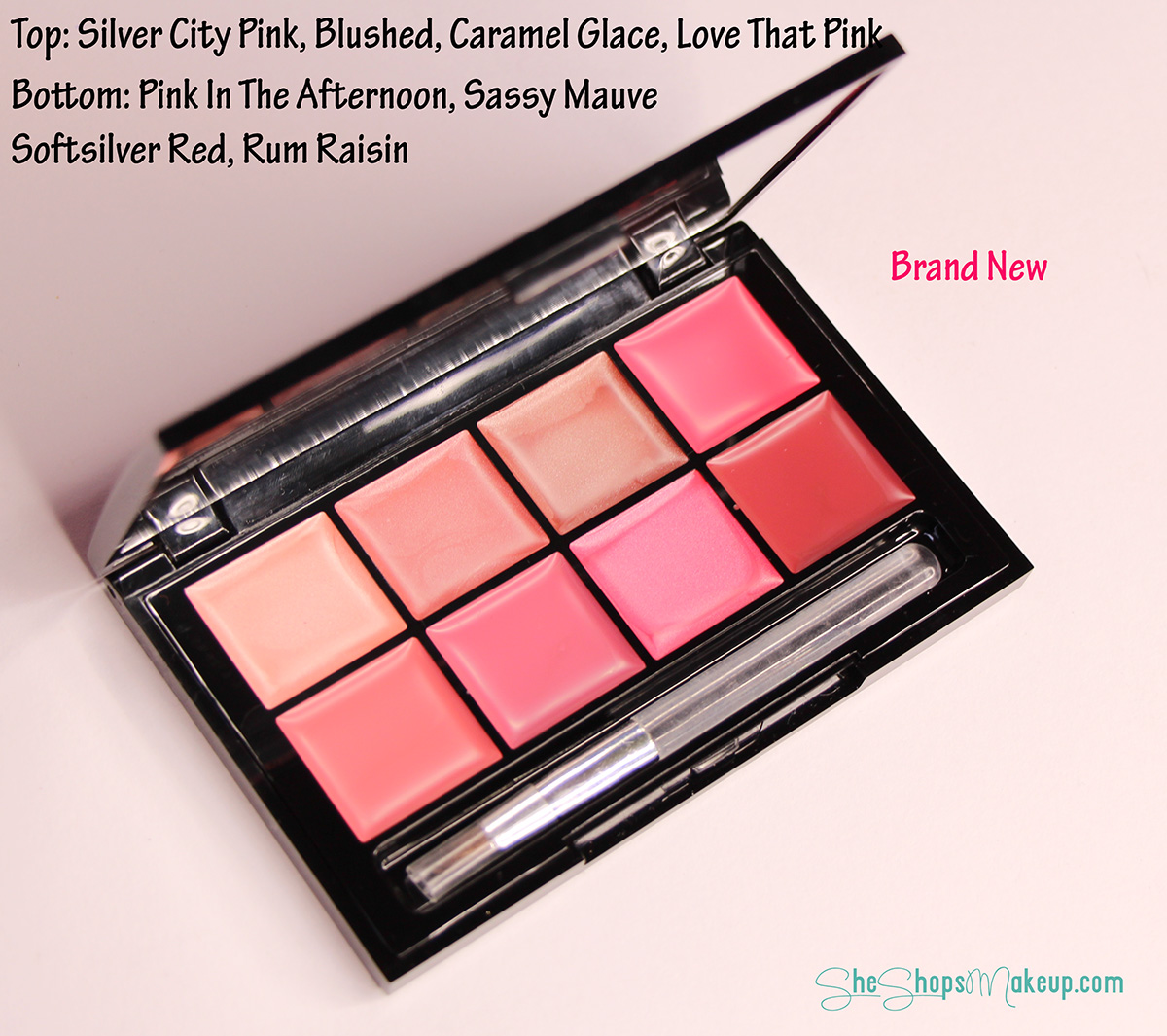The centerpiece of the image is a black makeup compact, opened to reveal eight shades of makeup in varying colors—primarily pinks and reds. The compact is slightly tilted to the right but remains centered in the frame. Inside the compact, a clear makeup brush is visible alongside a mirror on the left. The background is a blend of light pink, purples, and whites. Text overlays the image in different colors: black, green, bright pink, and lighter pink. At the top left, the text lists: "Top: Silver City, Blushed, Caramel Glaze, Love That Pink; Bottom: Pink in the Afternoon, Sassy Mauve, Soft Silver Red, Rum Raisin." To the right of the compact, in bright pink lettering, it reads "Brand New." The bottom right corner features the website "SheShopsMakeup.com." The overall style of the image suggests it is an advertisement for a makeup brand showcasing its diverse color palette.